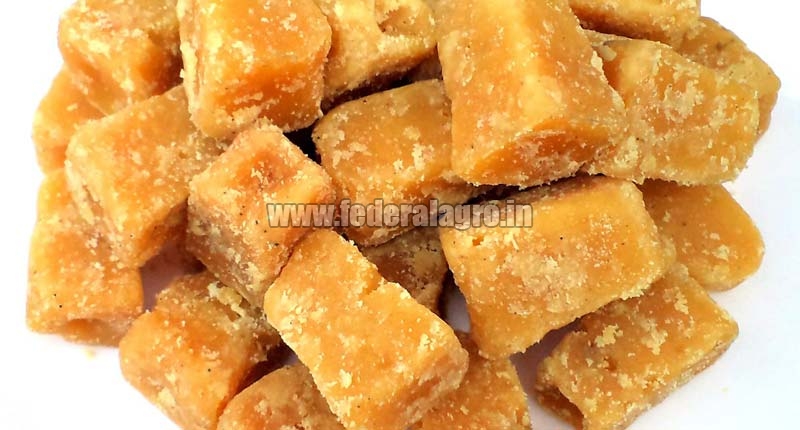This is a close-up photo of a small pile, approximately 20 pieces, of cuboid-shaped candies or food items. The items are deep orange to yellow in color, resembling caramel. Each piece is coated with sugar, evident from the tiny white flecks scattered across their surface. The pile is casually stacked with no particular order, and the cuboids are centrally positioned, dominating the image. The background is bright white, creating a stark contrast that highlights the food items. Across the middle of the image, there is a slightly transparent URL, "www.federalagro.in," written in white text with a transparent black background, adding a digital watermark to the photo.